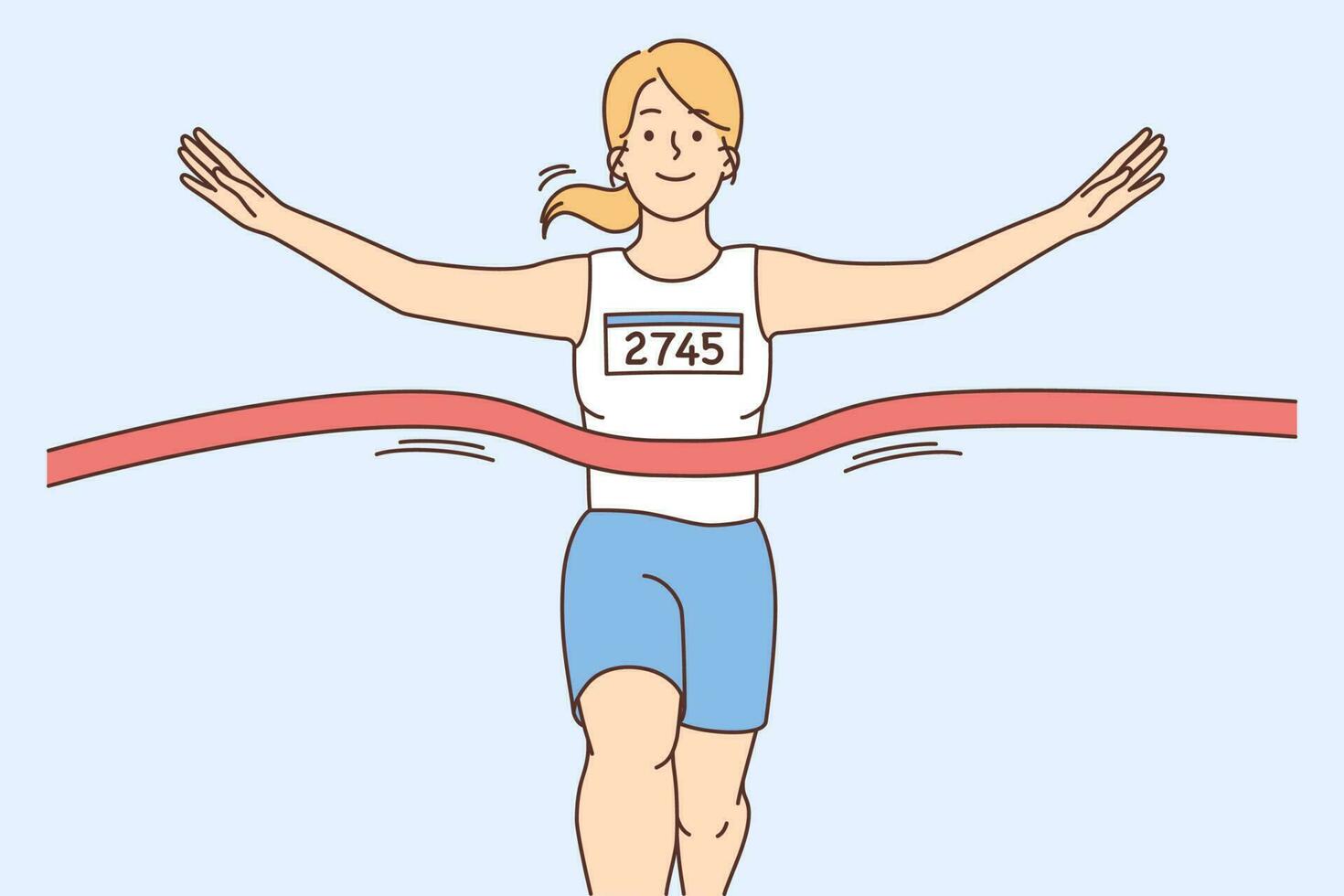The image depicts a simple digital drawing of a woman crossing the finish line of a race. The background is a solid light blue, emphasizing the central figure of the runner. She is a cartoon woman with a whitish complexion, smiling with a simplistic facial expression featuring dot eyes and a line smile. Her blonde hair is tied back in a ponytail. The woman wears a sleeveless white tank top with the runner's number "2745" displayed within a white box bordered at the top with a blue outline. She has on blue shorts that extend just above her knees. Her arms are raised, positioned at about 10 o'clock and 2 o'clock, as if celebrating her finish. The red finish line ribbon is wavy, indicating she has just broken through it, with action lines beneath it to emphasize movement. The image cuts off just above her ankles, leaving her feet unseen.